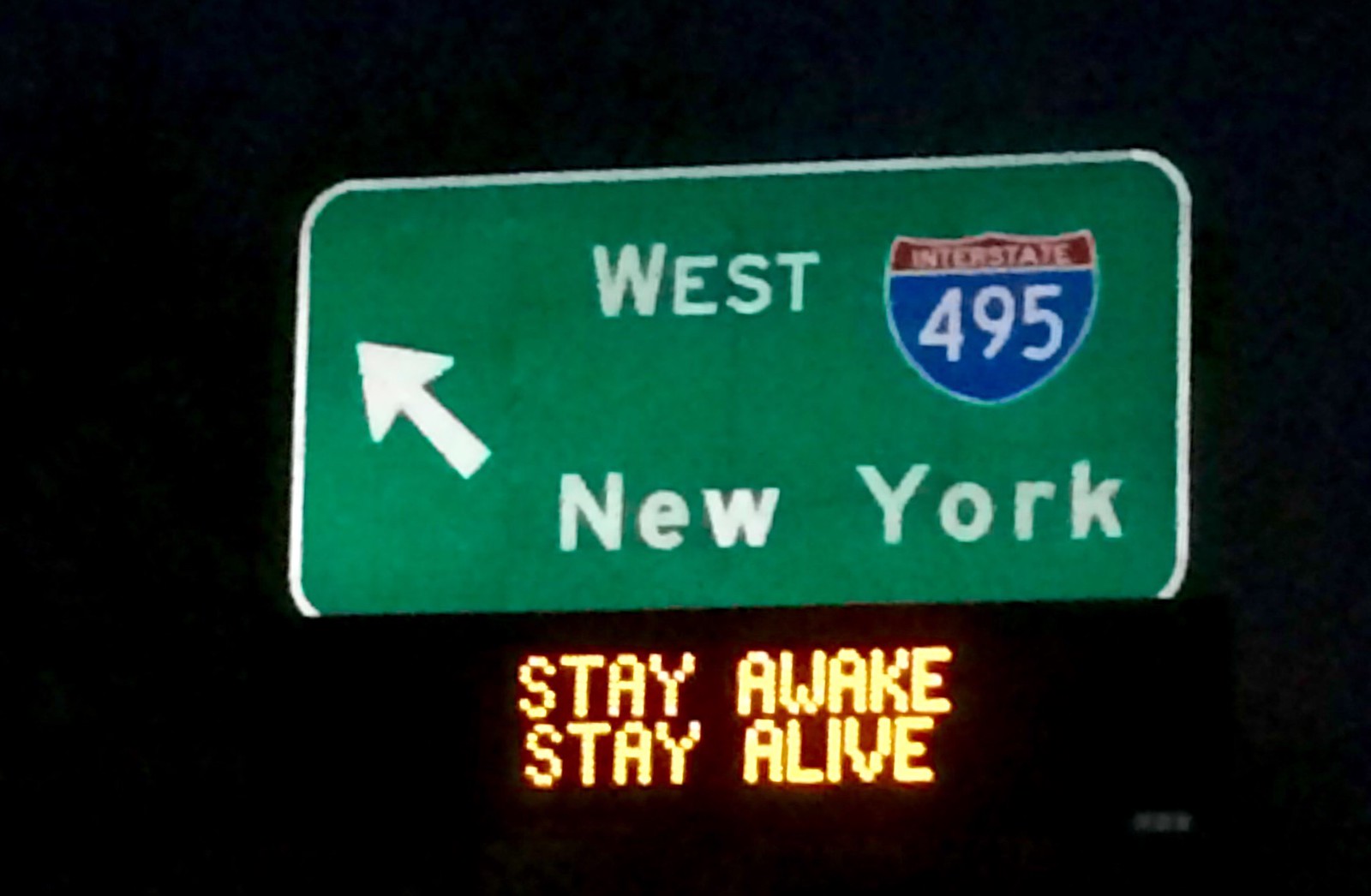In this nighttime photograph, taken from within a moving car, the pitch-black background accentuates a vividly illuminated green highway sign, creating a stark contrast. The sign is prominently displayed with a white border and bold white lettering that reads "West New York." Positioned at the top of the sign is a typical interstate shield, characterized by its red upper section and blue lower portion. This shield prominently features the number "495" in white, indicating Interstate 495. An arrow, pointing up and slightly to the left, directs drivers toward "495 West" bound for New York. Beneath this interstate sign, a digital message board emits a glowing amber hue with the cautionary slogan: "Stay awake, stay alive." The combination of these elements provides both directional guidance and a safety reminder for nighttime travelers.